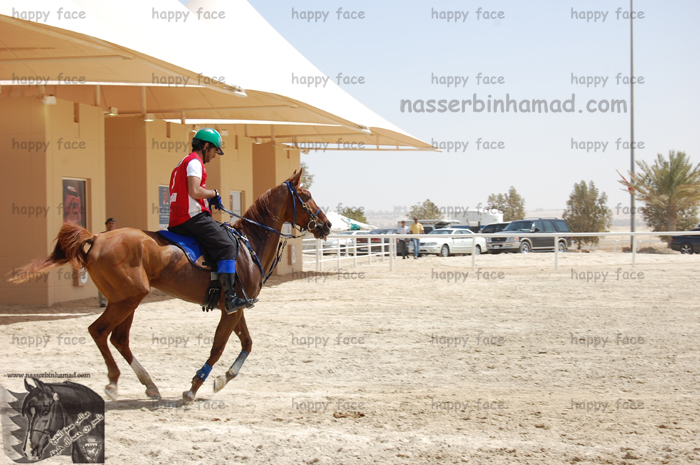In this detailed outdoor daytime photograph, a person is seen riding a trotting brown horse, adorned with a saddle. The rider wears a green equestrian cap and a short-sleeve red and white jersey, paired with gloves and black boots featuring a blue band. The background showcases a sandy dirt ground, flanked by a white fence and a parking area where two men walk in front of a black and a white car. A yellowish building with a white awning, possibly the horse’s stable, and a pole are visible behind them. Additionally, a graphic in the bottom left corner depicts a grey cylinder with banners beside a sketched horse. The sky above is light blue with scattered clouds. The image is marked with a repeating "happy face" watermark and a URL, "nasserbinhamid.com," in the upper right corner.